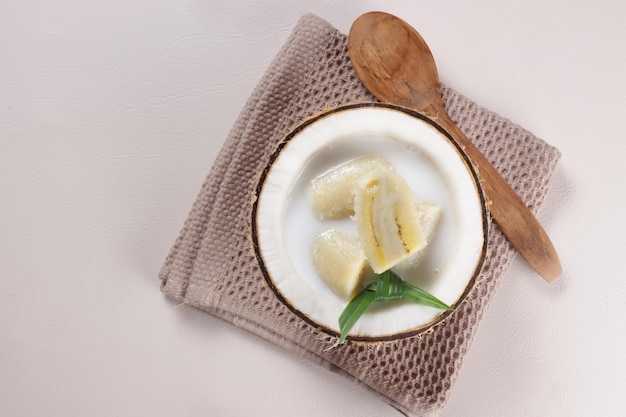The image showcases a meticulously arranged top-down shot of a food display on a plain white countertop. At the center, a small folded beige dish towel forms a neat square base. Resting atop this towel is a distinctive vessel that appears to be either a small white plate with a brown rim or possibly a halved coconut shell. Inside this vessel, quartered banana slices are arranged in a white liquid, likely coconut milk, accompanied by delicate white coconut flakes. Adding a touch of elegance, a green leaf, probably a banana leaf, is artfully tied into a decorative bow. To the right, a hand-carved wooden spoon lies beside the ensemble, creating a rustic yet sophisticated composition.